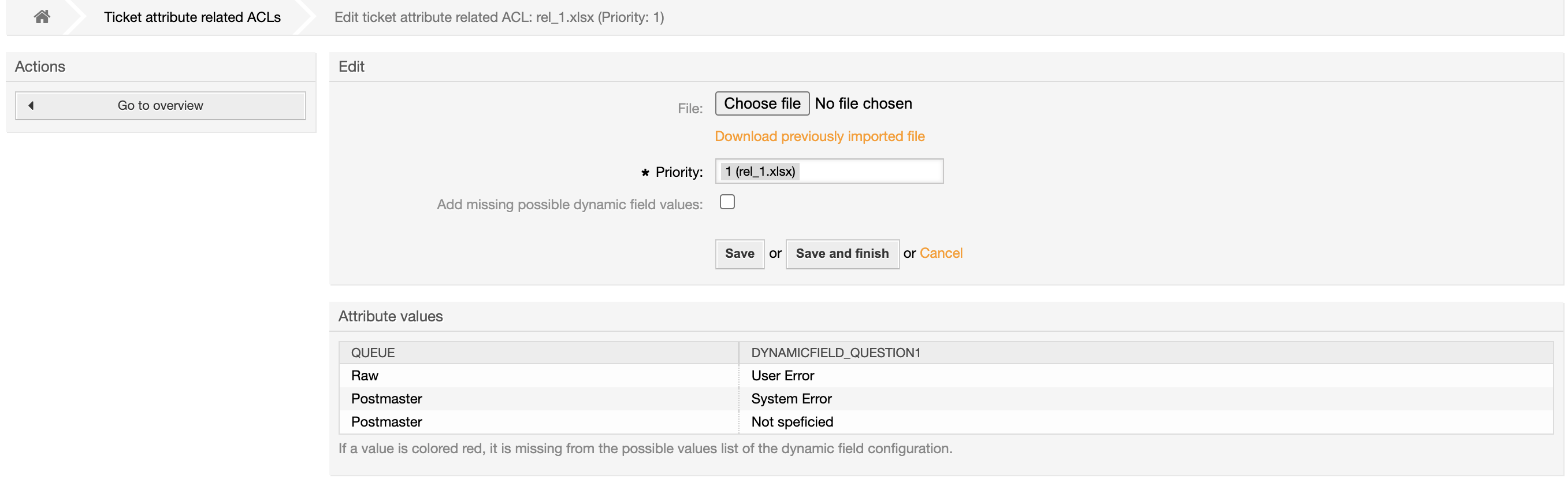The image is a horizontally rectangular screenshot of a user interface screen, possibly from a ticketing or task management system. In the upper left corner, extending across the top in a horizontal light gray banner, is a layout featuring multiple elements. 

On the left, there is a home icon. To its right is the label "Edit Ticket Attribute Rated ACL REL1.XISX Priority: 1." Beneath the home icon, there is a small gray box labeled "Actions," followed by a "Go to Overview" button. 

Adjacent to this, there is an "Edit" button next to a "Choose File" option displaying "No File Chosen," and another button offering to "Download Previous Imported File." The "Priority" field is visible, along with an input area for typing information. There is also an option labeled "Add missing possible dynamic field values" accompanied by an unchecked checkbox. 

At the bottom right of the interface, there are two buttons: one labeled "Save and Finish" and another "Cancel." The screen also references "Attribute Values Dynamic field," possibly indicating additional configurable options below the visible area. The overall design suggests a detailed form for editing and saving ticket attributes.